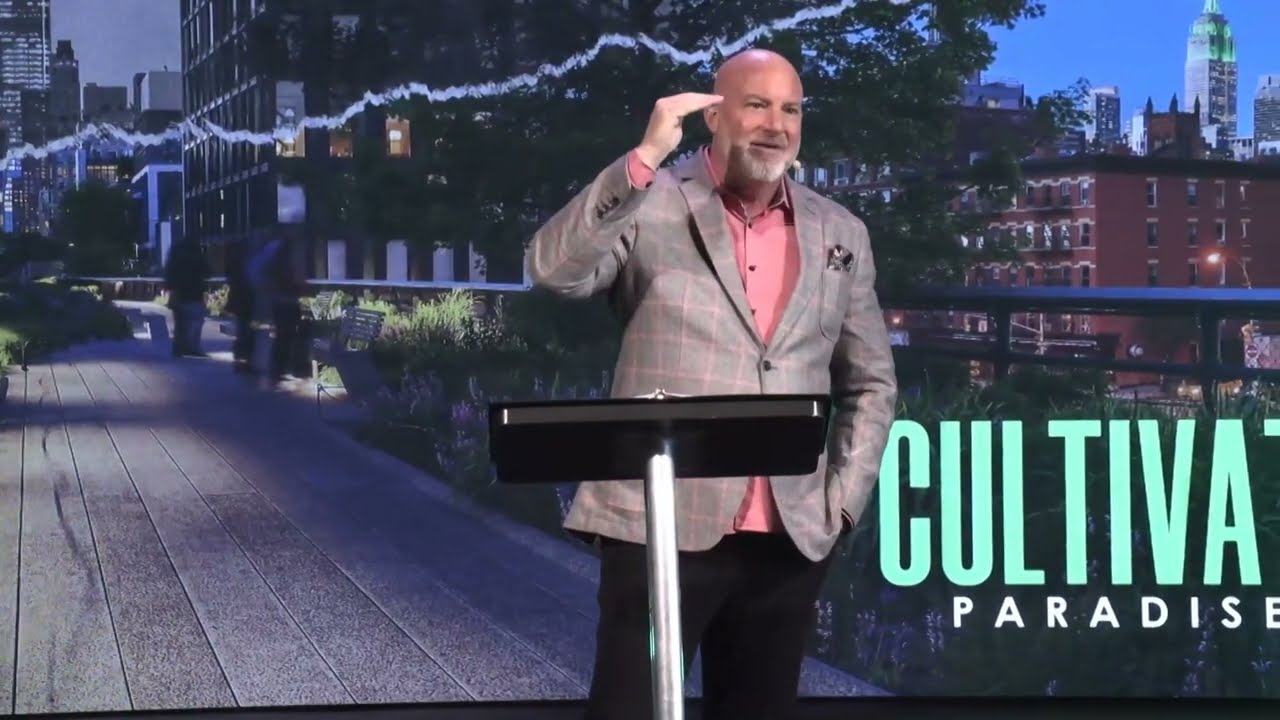The image features a man giving a speech at a podium. He is shown from the knees up, wearing a stylish gray and pink checked blazer over a pink shirt, with black trousers. The man is bald and sports a white-gray beard and glasses. His left hand is casually placed in his pocket, while his right hand is raised to his eyes, gesturing expressively as if to emphasize a point. The podium itself has a black angled top and a silver cylindrical stand, with a binder visible on it.

Behind the man is a large mural or screen, depicting an urban park or garden walkway complete with benches, lights, and lush greenery, all set against a cityscape in what appears to be New York City. Notable landmarks include the Empire State Building and typical New York row houses. In the bottom right of the backdrop, the phrase "Cultivate Paradise" is prominently displayed, partially obscured but legible in large green and smaller white letters. This background suggests the man might be presenting on urban development or park planning initiatives.